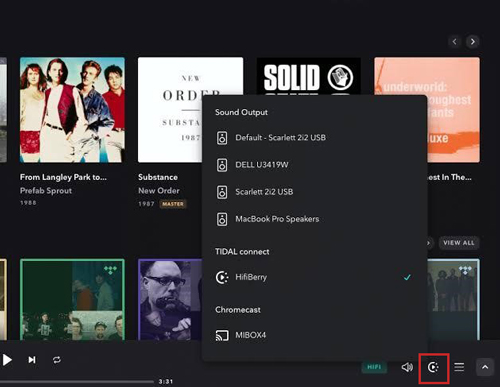The image features a screen with a black background, showcasing a collection of media and audio settings. 

At the top, there are four images displayed side by side:

1. The first image on the top left depicts four Caucasian individuals—three males and one female. Beneath the image, the text reads "From Langley Park to Prefab Sprout."
2. The second image is a white square with the text "New Order, Substance, 1987." Below the square, the text repeats as "Substance, New Order, 1987."
3. The third image is a black square with the word "Solid" in white text, followed by a pink square with "Underworld."
4. The fourth image contains a square with four smaller squares inside it, three of which include tiny photos of individuals.

Across the bottom, there are partially visible images, including:

1. A purple background with four small photos of various individuals.
2. A large black box with white text listing audio settings from top to bottom: "Sound Input, Default Scarlett 212 USB, Dell U3419W, Scarlett 212SB, MacBook Pro Speakers, Tidal Connect, HiFiBerry, Chromecast," and "MIBOX4."

This caption provides a detailed description of the screen's layout and content.